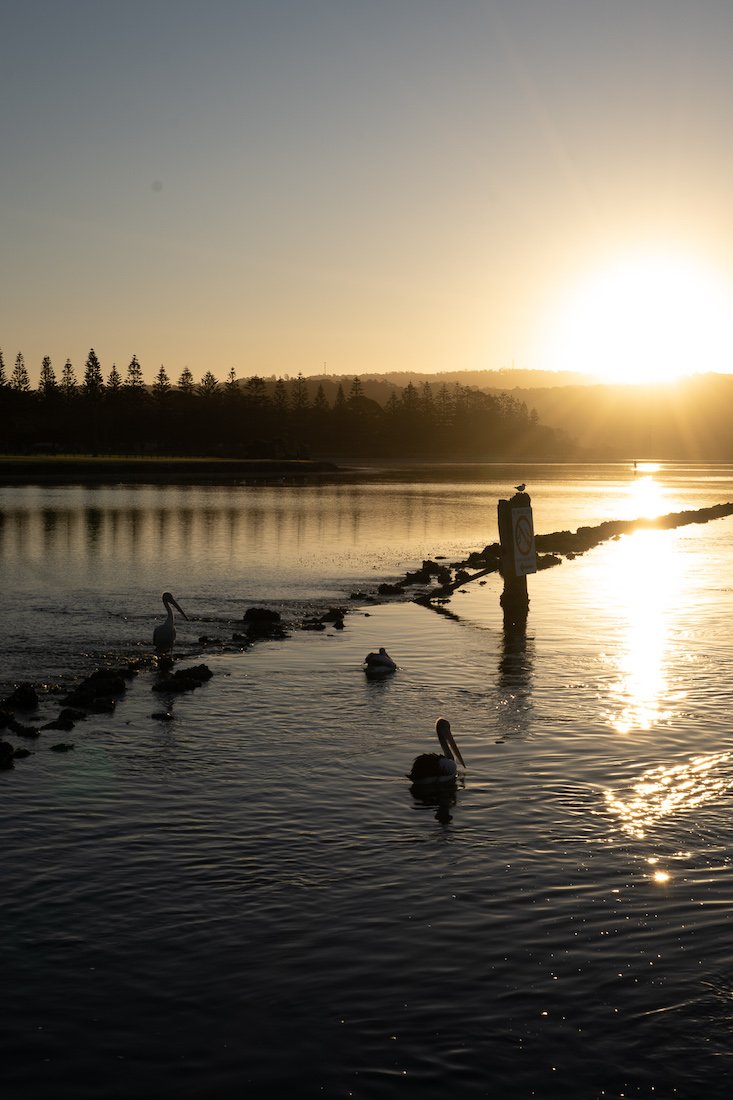A serene lakeside scene captures the moment the sun is setting, casting a gradient from deep blue at the top of the sky to warm orangey pink near the horizon. The bright sun peeks over distant hills, its golden reflection stretching across the dark, shimmering surface of the lake. Three pelican-shaped waterfowl, with their distinctive long bills, can be seen swimming on the water, with one bird silhouetted against a rock towards the left. A "no" sign with a red circle is prominently placed in the lake, bearing a sparrow perched atop it. In the background, a tree-lined mountainous range creates a picturesque boundary to this tranquil setting.